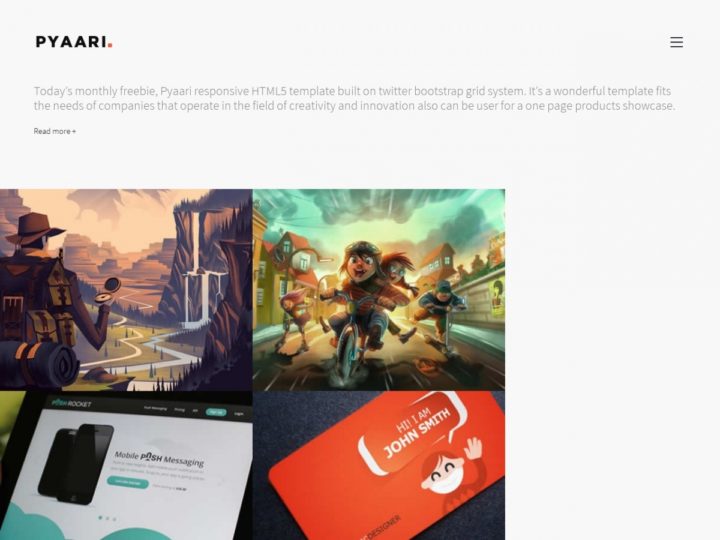In the upper left corner of the image, the text "PYAARI" is prominently displayed in bold black uppercase letters, followed by a red period for punctuation. Below this, the phrase "Today's Monthly Freebie" introduces the featured item: the PYAARI responsive HTML5 template, which is built on the Twitter Bootstrap grid system. The description highlights that this versatile and impressive template is ideal for companies in creative and innovative fields and is also suitable for one-page product showcases. 

A call-to-action to "Read More" is positioned underneath, inviting further engagement. Below this section, there are four distinct squares, each showcasing different animated scenes:

1. The first square features an animated explorer wearing a cowboy hat with a compass in hand. The explorer stands before a vast, tall valley surrounded by brown mountains and scattered trees.

2. The second square depicts animated young characters enjoying a day out. Some are riding scooters, while two children in the middle are on a bicycle, their faces lit up with excitement, mouths open, and eyes wide.

3. In the lower left corner, there is the phrase "Mobile Messaging" accompanied by an image of a smartphone screen.

4. The final square on the right presents an orange credit card with the text "Hi, I’m John Smith" and features an animated character wearing a mask and waving.